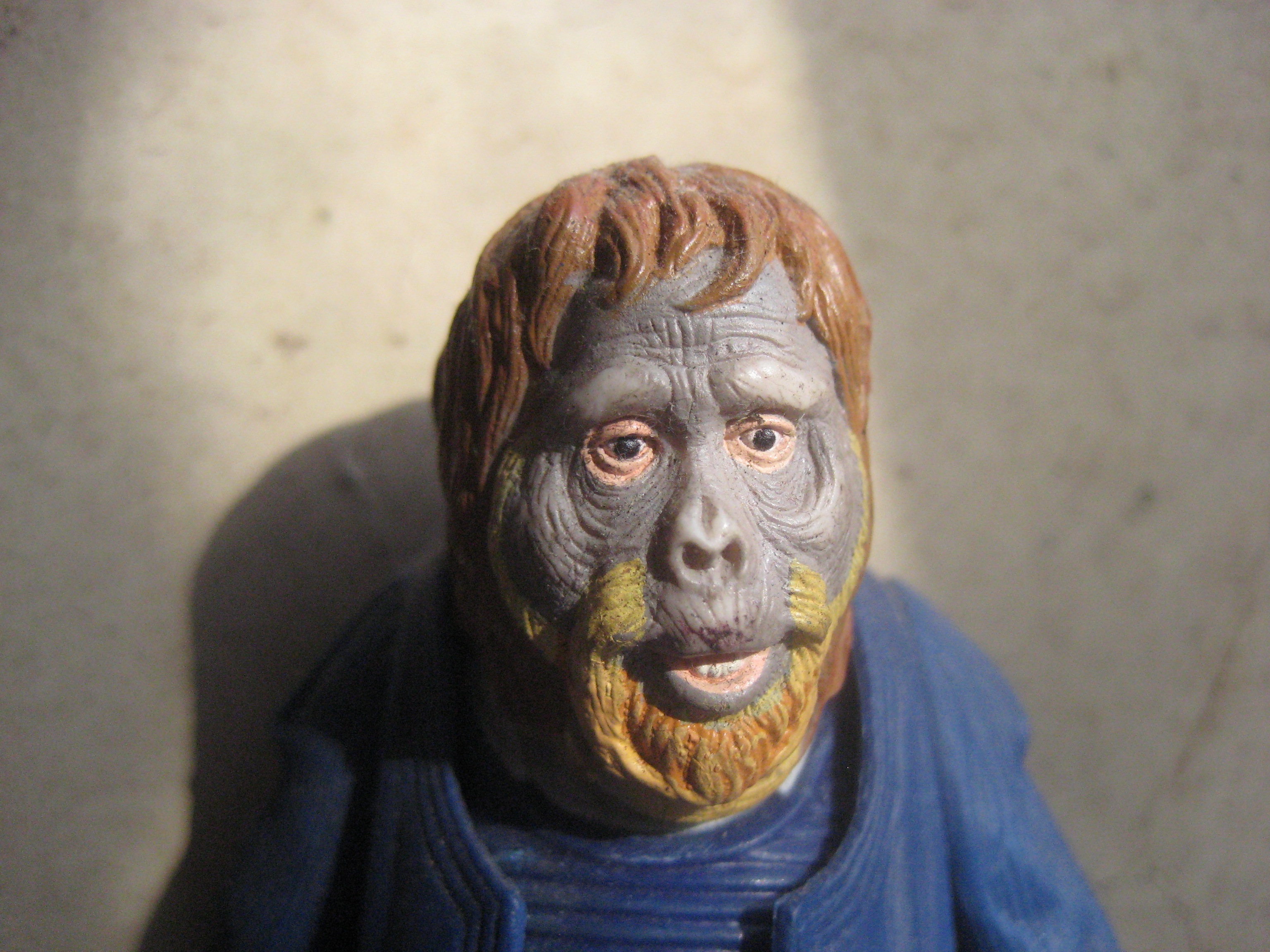The image depicts a highly detailed figurine central to the composition, reflecting a character from the "Planet of the Apes" movie. The figure has distinct features: a hybrid ape-human face with gray, wrinkled skin except for the area around the black eyes and mouth, which has a human-like white skin tone. The character is adorned with medium-length brown hair and a noticeably two-toned beard that is predominantly blonde with hints of orange or brown. The attire is a blue shirt, complemented by a blue jacket. The backdrop is a plain, white or cream-colored wall, casting a shadow that emphasizes the figure's prominence. The photograph captures the essence of the figurine, showcasing its intricate design and the contrast between its human and ape characteristics.